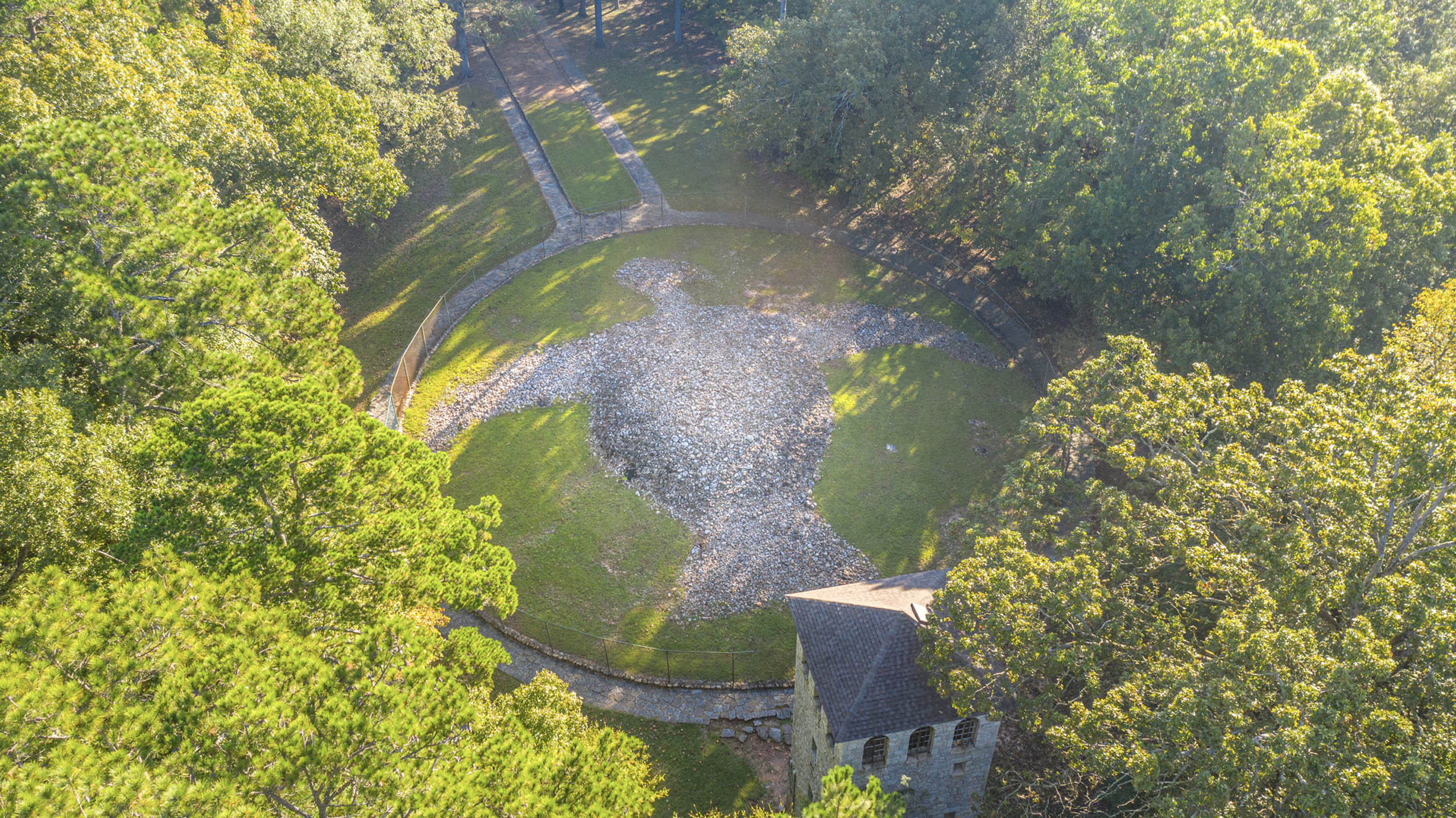This is an overhead outdoor image featuring a sunlit landscape with light from the sun illuminating the scene, though the sun itself is not visible. The image is framed by lush, green decidious trees on both the left and right sides. At the center of the scene is a prominent green hill encircled by a gray gravel pathway, which extends outward in two straight, slightly left-angled paths at the top of the hill. At the bottom of the hill is a tall, stone tower with a dark gray, four-sided pyramidal roof and three windows at the top.

Centrally located on the green hill is an intricate gray bird pattern, artistically made from gray rocks or gravel, featuring two wings, a tail, a rounded body, and a curved beak facing to the right. The gray paths and bird-like pattern create a striking contrast with the green surroundings. Surrounding this elaborate display are expanses of verdant deciduous trees, adding to the scenic beauty and creating a harmonious natural frame around the architectural and artistic elements in the image.